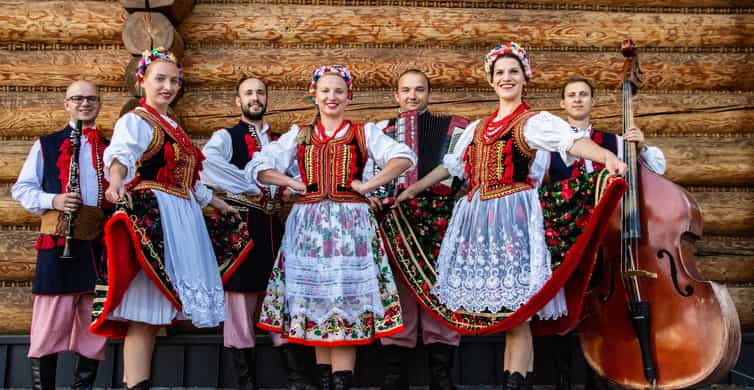The image features a group of seven people dressed in intricate folk attire, suggestive of traditional costumes from regions such as Lapland or the Netherlands. The front row consists of three women, each wearing a flower crown atop their heads, with ornate red vests over white shirts, and skirts featuring vibrant floral designs on a white background. Their outfits are accented with stripes in red, yellow, and black. The women are all smiling and sporting black boots.

Behind the women are four men, each donning baggy pants tucked into black boots and long blue shirts that extend to mid-thigh, adorned with red ruffles. The men are also smiling, adding to the lively and cheerful atmosphere of the group.

On the far left of the image, a bald man with glasses, likely part of the musical ensemble, holds a clarinet. To his right, a woman stands with her body slightly turned but face towards the camera. Centrally situated is a woman with her hands on her hips, directly facing the viewer. In the background, a man is seen holding an accordion. Further to the right, another woman faces the camera, and finally, on the far right, a man holds an exceptionally large, dark-wood cello that towers over him, suggesting a whimsical touch to the composition. The backdrop appears to be a rustic log wall, enhancing the traditional and folkloric essence of the scene.